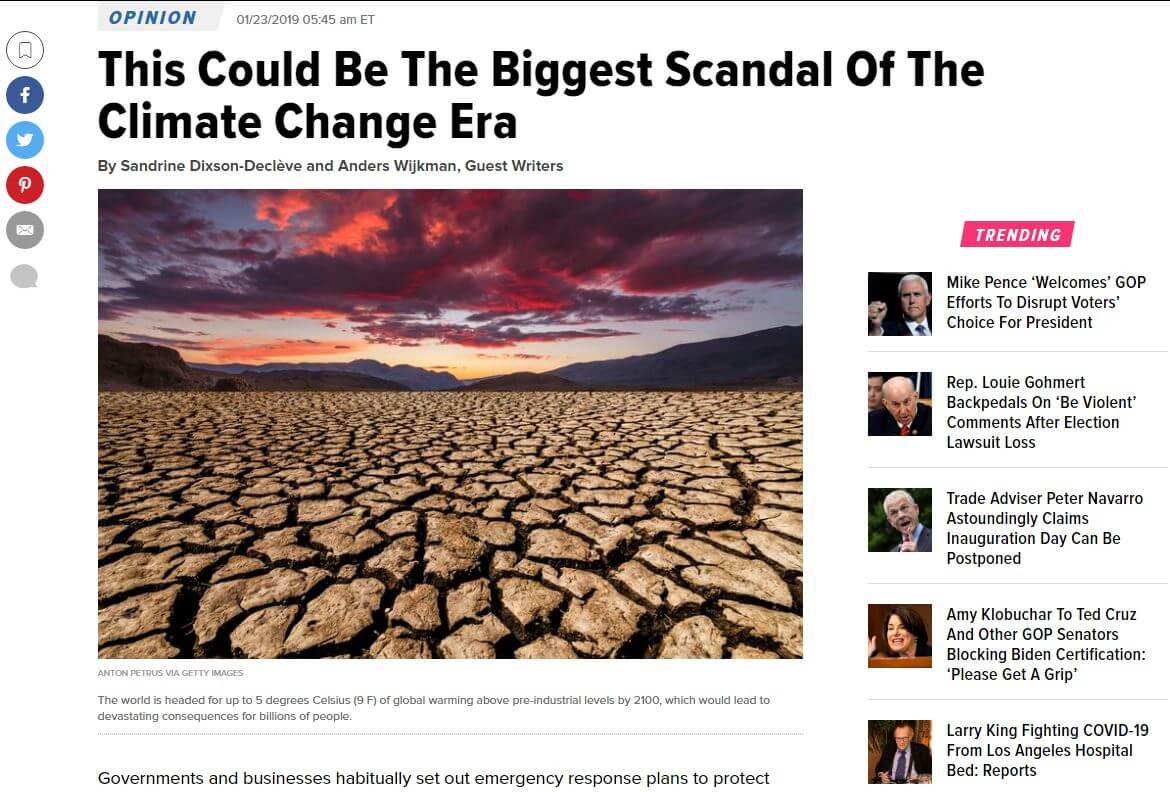This detailed caption describes the screenshot of a webpage taken from a site that could be a news outlet or blog. Centered at the top is a gray box labeled "Opinion" in blue font. To its right, the date and time are displayed as "01-23-2019, 05:45 a.m. ET." Adjacent to these details, a vertical white column features various circular icons for bookmarking, sharing on Facebook, Twitter, Pinterest, emailing, and another icon resembling a thought bubble, likely for text or general sharing.

Prominently positioned is the headline, “This could be the biggest scandal of the climate change era,” authored by guest writers Sandrine Dixon de Cleve and Anders Wickman. Below the headline, a striking image dominates the page, depicting a dramatic scene with a dark, ominous red sky occupying the upper half and cracked, arid ground resembling a desert landscape extending from the foreground to the background.

Overlaying the image is a bold text stating, “The world is headed for up to 5 degrees Celsius of global warming.” On the right side of the page, additional articles are listed, offering clickable links for further reading.